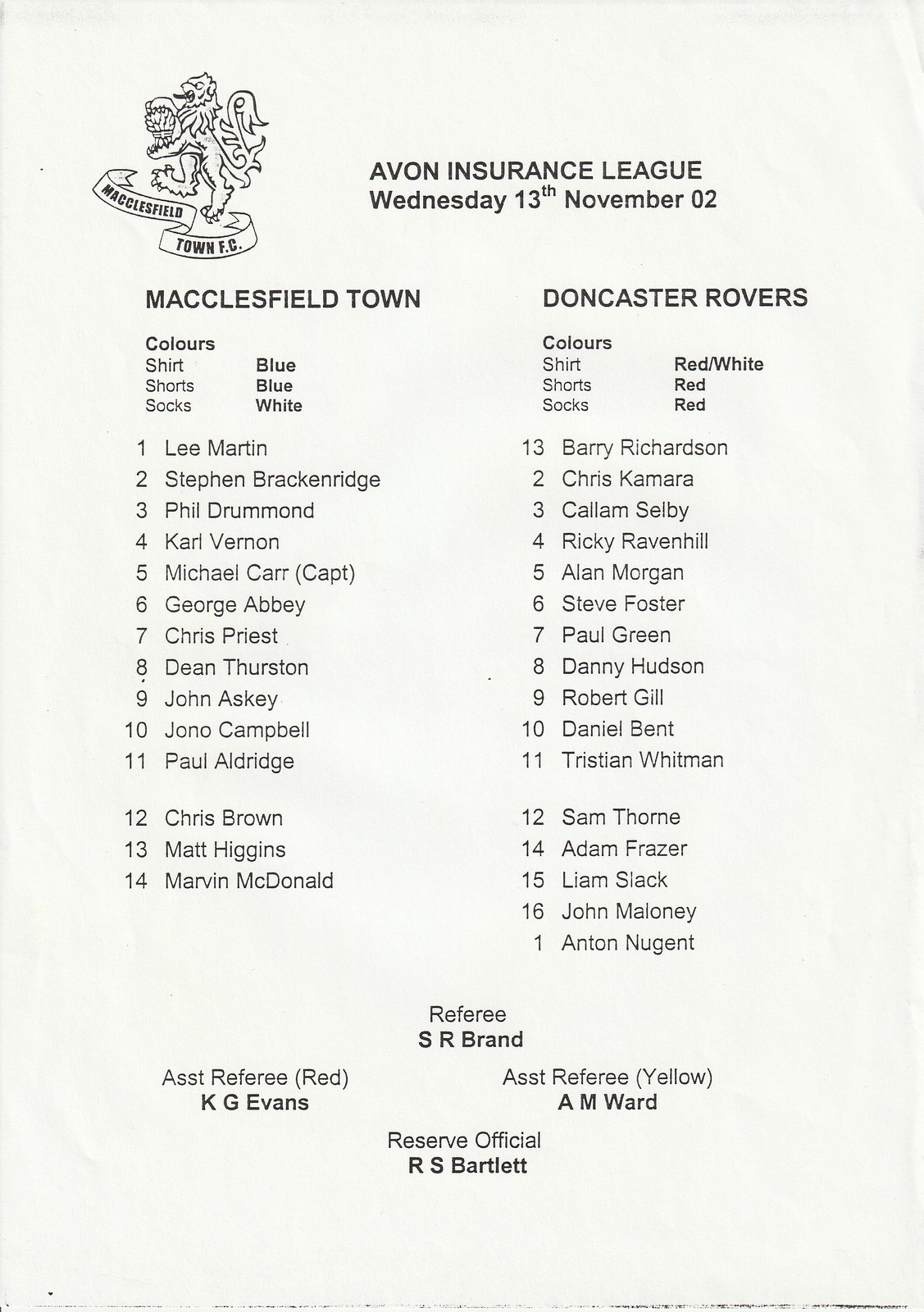This image is a detailed page from a soccer program or magazine, predominantly white with black text. At the center top, it features a heading: "Avon Insurance League, Wednesday, 13th November 2002." The upper left corner showcases a regal lion logo with a ribbon below that reads "Macclesfield Town FC." Below this, the roster for Macclesfield Town is listed, detailing their uniform colors: blue shirts, blue shorts, and white socks, followed by a list of 14 players. On the right side, the column for Doncaster Rovers lists their colors: red and white shirts, red shorts, and red socks. Their team roster appears somewhat disordered, listing 17 players. At the bottom of the page are the names of the match officials: Referee S.R. Brand, Assistant Referee K.G. Evans (in red), Assistant Referee A.M. Ward (in yellow), and Reserve Official R.S. Bartlett.